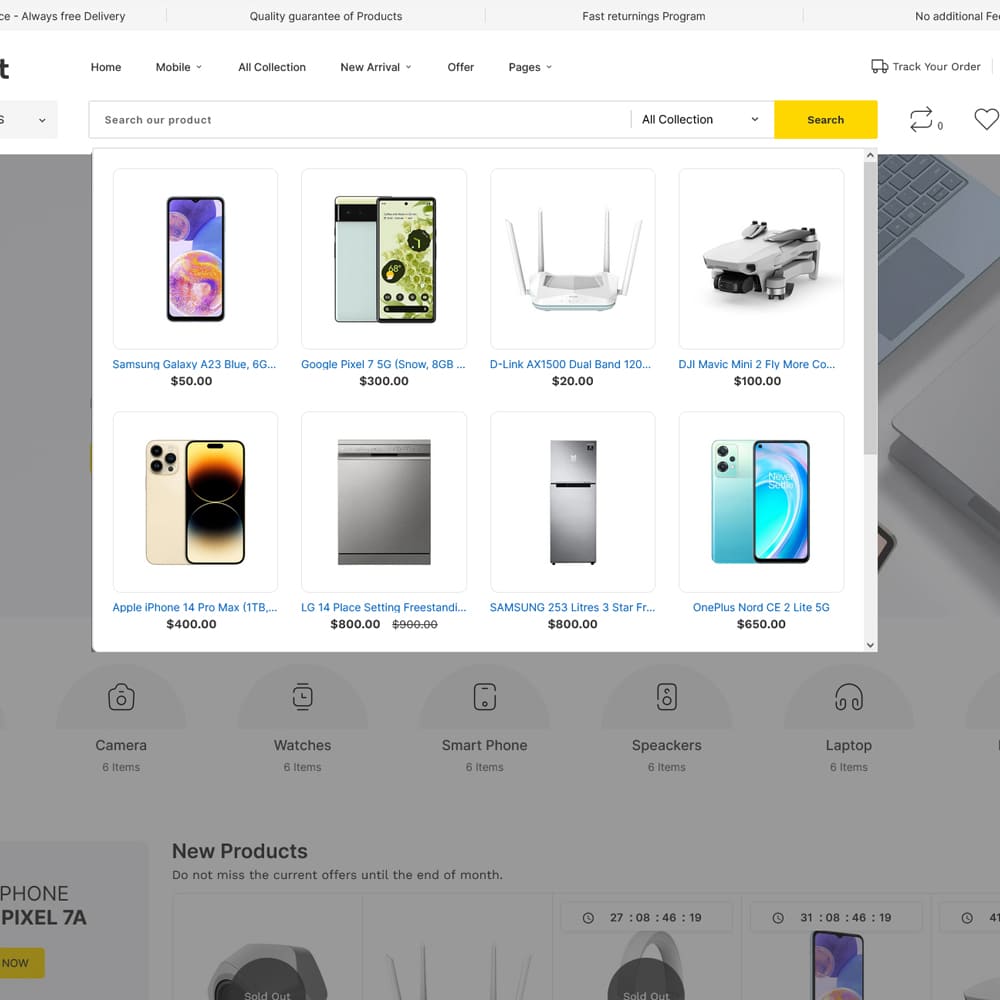Cropped webpage screenshot showcasing a shopping interface. At the top, a grey banner prominently displays partial promotional text: "Quality, guarantee of products, fast returnings program, no additional…" Dissected further below, the white header lists navigational categories: "Home, Mobile, All Collection, New Arrival, Offer, and Pages," with a "Track Your Order" option situated on the far right. Centrally positioned at the bottom of this header is a search bar labelled "Search our product." Adjacent to this, a dropdown menu pre-selects "All Collection," followed by a yellow search button.

Directly beneath the search bar, a dropdown menu reveals eight product thumbnails, arrayed in two rows of four. Each item displays a visual preview, with a scrollbar on the far right for further navigation.

In the webpage background beyond the primary content, additional categories like "Camera, Watches, Smartphones, Speakers, and Laptop" are partially visible at the bottom.